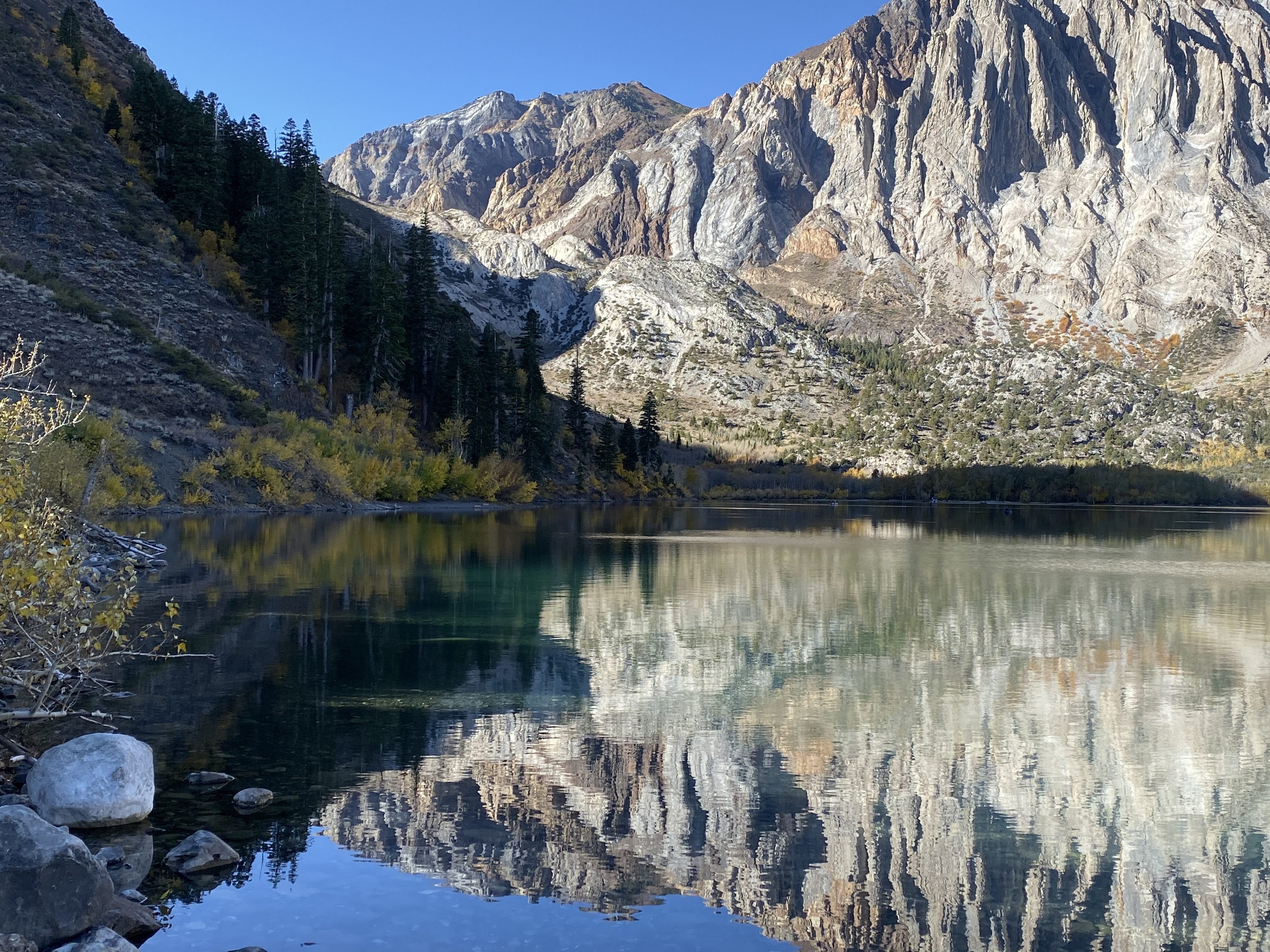The image captures a serene outdoor scene during the daytime, dominated by a large, tranquil lake stretching from left to right. The water in the lake is mostly still with slight ripples, subtly distorting the reflections of the towering gray and brown mountains that surround it on both sides and in the distance. On the left-hand side of the image, the mountains showcase an array of green, yellow, and orange plants climbing their slopes, amidst scattered darker rocks and some bushes near the shore. A small row of dark green trees can be seen ascending one of the mountains, casting shadows. The sky above is a clear, vivid blue, unmarred by any clouds. Additionally, the bottom left corner of the picture features a handful of large rocks, adding texture to the otherwise smooth shore where the photographer presumably stood.